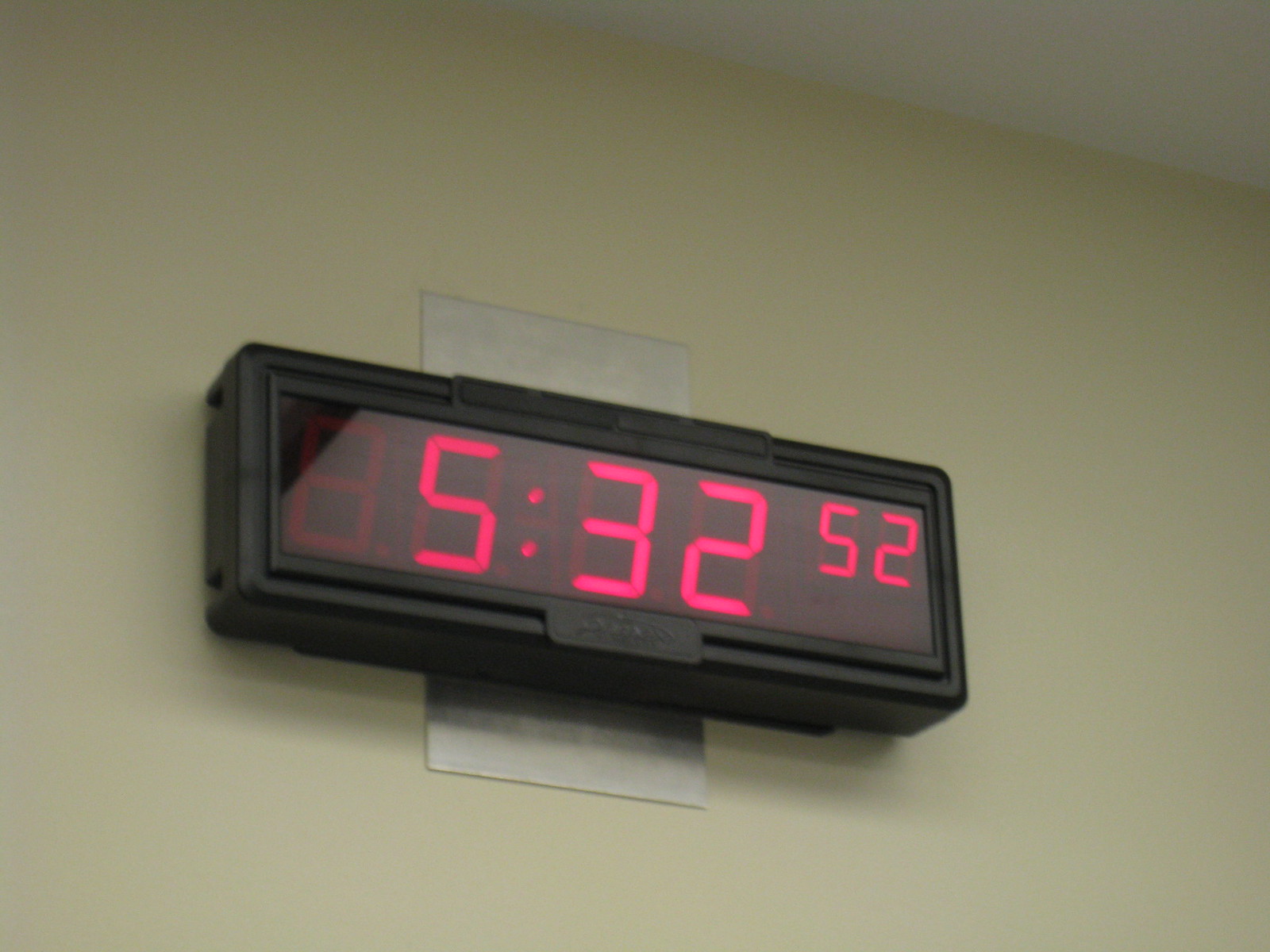This close-up image captures a digital clock mounted on a vertically oriented rectangular metal plate, affixed to a cream-colored plaster wall. The clock itself features a rectangular black frame, encasing a digital display with vivid red numbers. The time reads 5:32, with the seconds marked at 52 in the top right corner of the clock face. In the upper right of the image, a portion of the white ceiling is visible, adding depth to the setting.